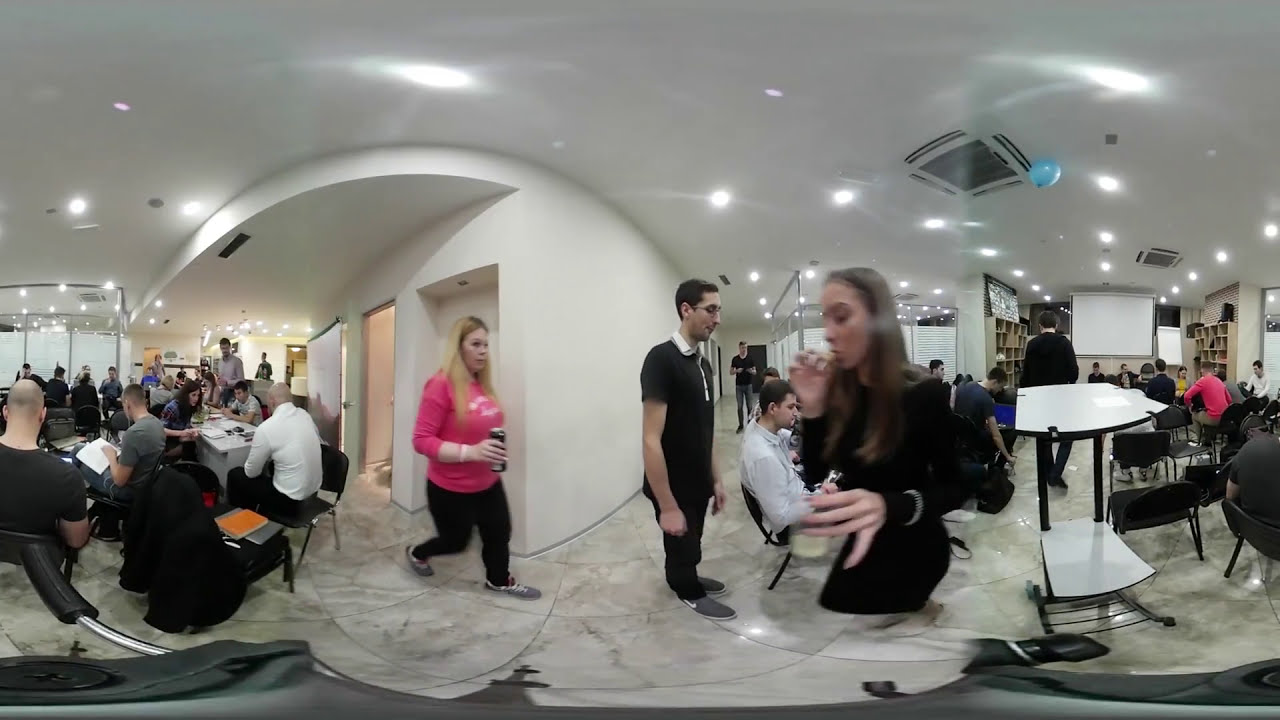The image showcases a spacious, modern room, possibly a library or a casual meeting area, characterized by its white walls and ceiling adorned with circular lights arranged in horizontal rows. The light gray tile floor complements the minimalist design, dotted with white and black tables. People are scattered throughout the room, predominantly seated and engaged in reading, with a woman crossing the room from left to right holding a dark-colored cup. A man stands in the center, surveying his surroundings, while another woman is seen eating as she moves from right to left. The left side of the room features an elevator. The atmosphere is professional yet relaxed, evocative of a business environment taking a casual break, with individuals dressed in work attire—shirts in white, gray, black, blue, and tan. The scene also includes a variety of activities around these tables, such as light discussions and solitary reading. The ceiling vents are a darker shade, and windows line the left wall, contributing to the bright ambiance of the room.